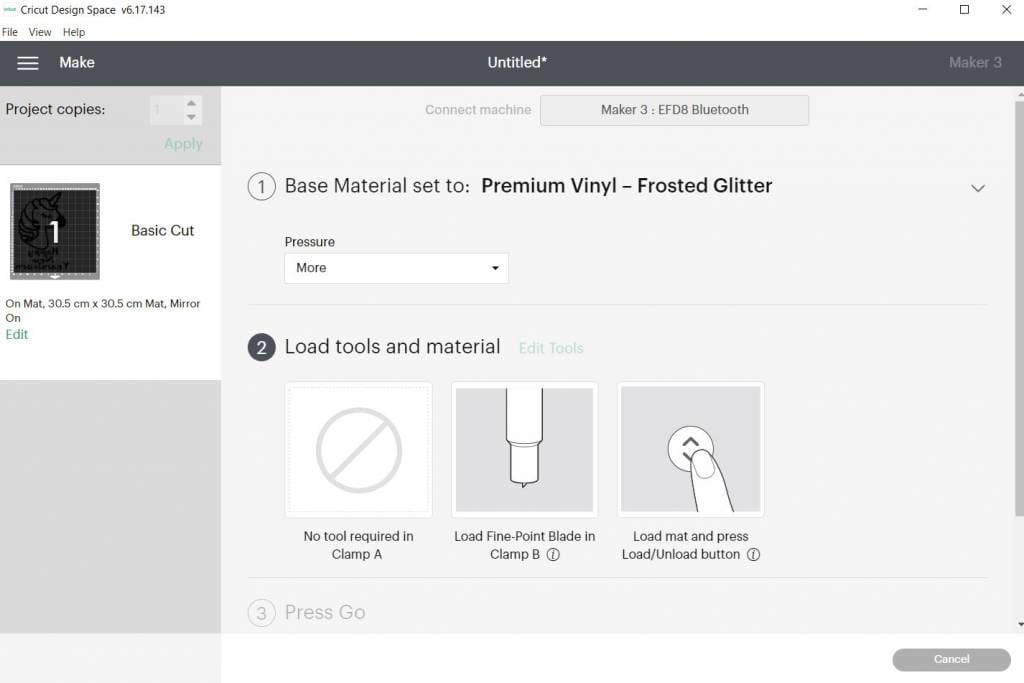This is a detailed screenshot of the app Circuit Design Space v6.17.143. 

**Header and Navbar:**
- In the top-right corner are the three standard window control buttons: close, minimize, and full screen.
- The upper left features options labeled: File, View, and Help.
- Below these options is a dark gray bar highlighting an untitled project, denoted by an asterisk.

**Sidebar and Menus:**
- On the left, a vertical gray menu begins with an icon of a hamburger menu followed by "Make."
- Further down, the menu reads "Project Copies" with a grayed-out number selector to its right. Below this, there is a green "Apply" button.
- This vertical sidebar is intersected by a white horizontal bar.

**Primary Workspace:**
- Beneath the white bar, there's a black section featuring a large "1" and the label "Basic Cut." Details include "on mat 30.5 cm x 30.5 cm mat, mirror on," along with a green "Edit" button.
- In the primary field, at the top-right, it reads "Connect Machine" next to a peach-colored field displaying "Maker 3; EFD8" and "Bluetooth."

**Materials and Tools Setup:**
- Underneath, there's a section with headers encircled by numbers. Header "1" sets the base material to "Premium Vinyl - Frosted Glitter" alongside a dropdown menu for "Pressure."
- Below this, section "2" involves loading tools and materials. It contains three graphical icons:
  - A crossed-out circle labeled "No tool required in Clamp A."
  - An image that looks like a pen or knife with the text "Load fine-point blade in Clamp B" and an italicized 'i' in a circle for more details.
  - A finger pressing an up/down button captioned "Load mat and press load/unload button," also with an information icon.

**Final Steps:**
- Step "3," which reads "Press Go," is grayed out, with a gray "Cancel" button located in the bottom right, featuring white text inside a gray capsule.